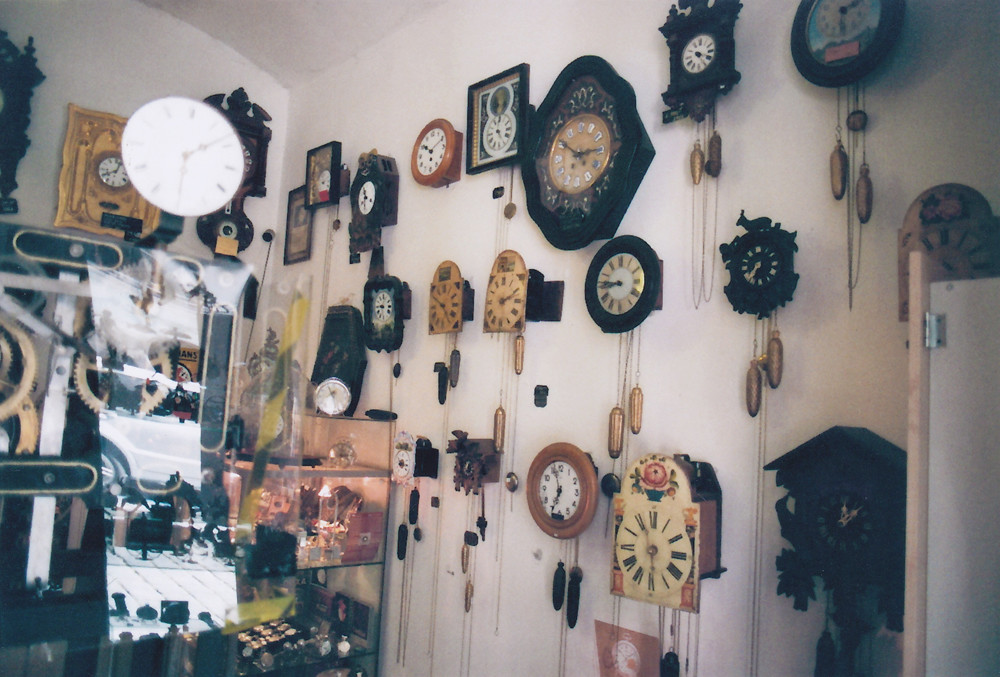The indoor photograph showcases a room with white walls and a white ceiling, adorned with an impressive assortment of antique clocks on both the right and left walls. There appear to be approximately 20 clocks, varying widely in size, shape, and style, predominantly featuring wood-tone or black finishes. Many of the clocks exhibit long pendulums or chains with hanging chimes, and most have their hands set to different times, contributing to a chaotic yet captivating display of timepieces. In the bottom left corner of the image is a glass display case containing various knick-knacks, stopwatches, and unidentified objects, enhancing the room’s antique charm. A clear device with visible gears also sits on the left, further emphasizing the collection's vintage theme. Overall, the room resembles an antique store, teeming with historical allure despite the arguably unattractive appearance of the clocks.